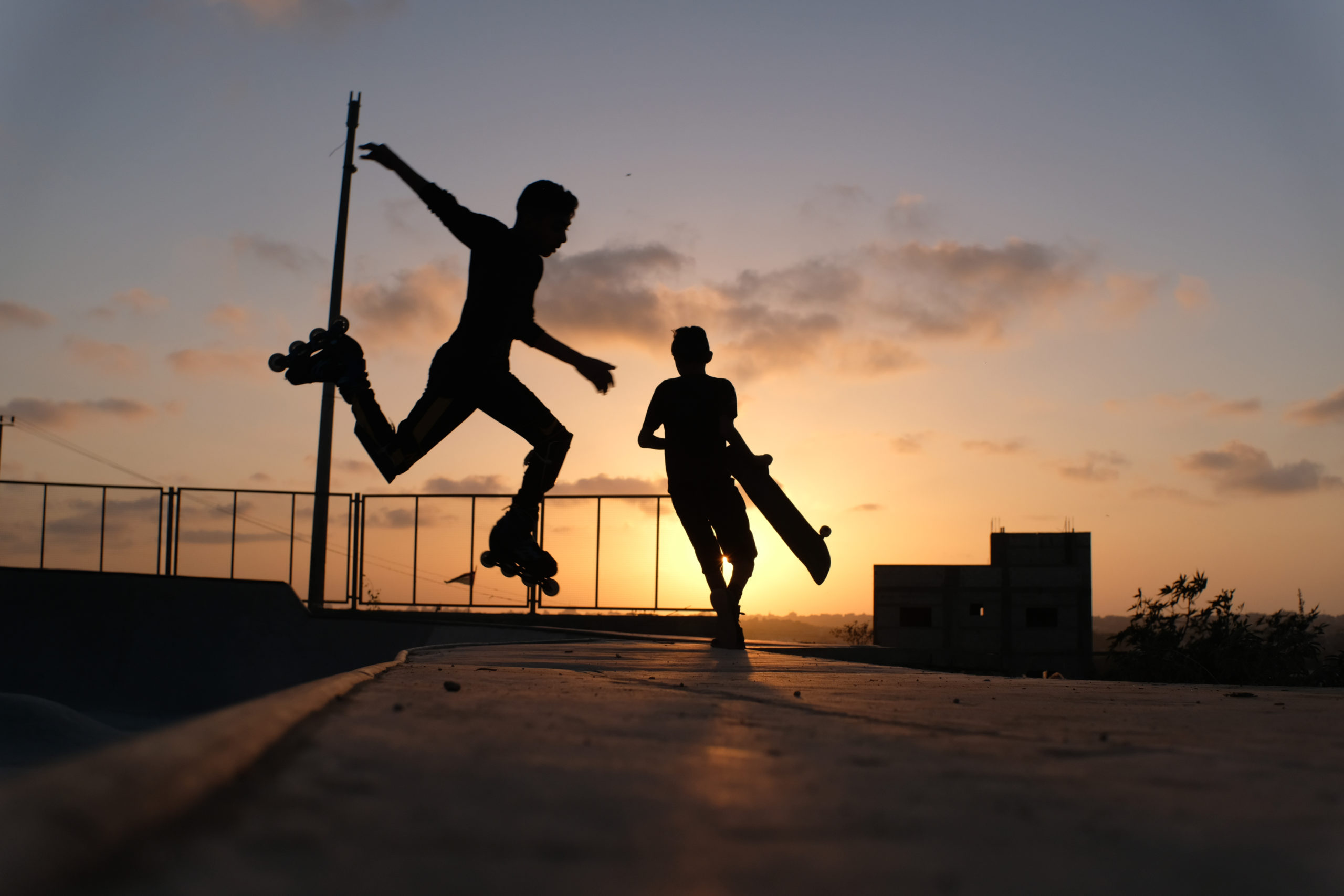In the midst of a vibrant sunset sky painted with hues of orange, blue, and gray, a photograph captures the dynamic silhouettes of two boys at a skate park. The boy at the center of the image is airborne, arms raised, showcasing his roller skates with their distinctive four wheels illuminated by the setting sun behind him. Beside him, another boy holds a skateboard in his left hand, seemingly caught in mid-stride, giving the impression he is running. The black figures of these boys stand out against the glowing sky, highlighting their energetic movements. They are situated on cracked concrete, with a backdrop featuring a fence to the left and a building to the right. Further in the distance, faint silhouettes of trees are visible, adding depth to the scene. The image, free of any text or identifying markers, powerfully conveys the essence of youthful exuberance in an evening skate park setting.